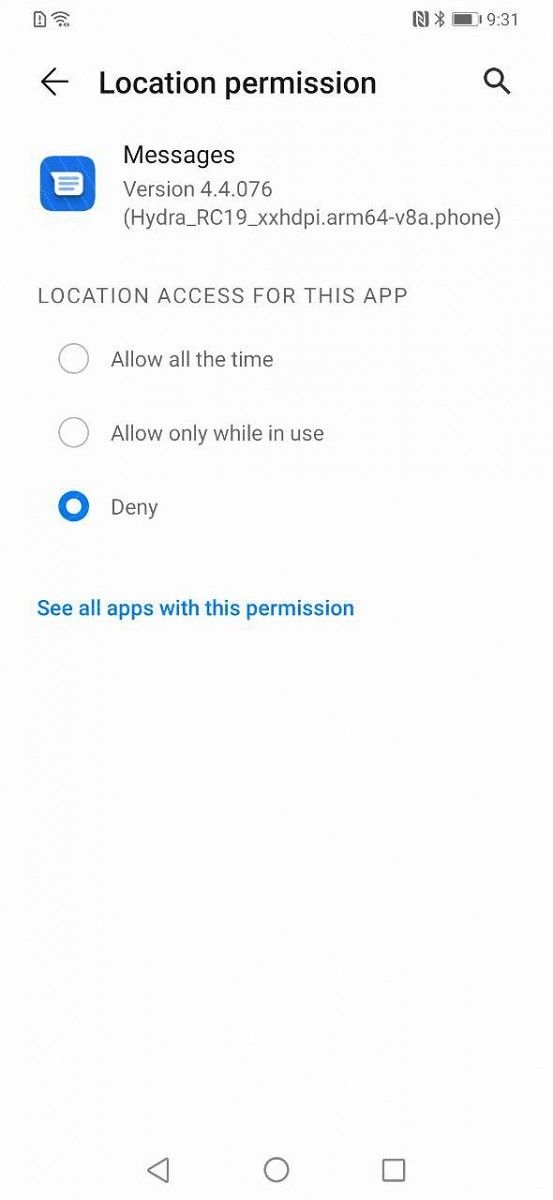The screenshot, captured in portrait mode, features a predominantly white background that is slightly darker than the rest of the screen. In the upper-left corner, an exclamation point is enclosed in a shape, while the upper-right corner displays the time as 9:31 and a battery level of approximately 60%. Below this, there is a bold back arrow next to the heading "Location Permission," followed by a search icon.

Further down, an icon representing messaging is displayed alongside the text "Messages Version 4.4.076." A section titled "Location Access for this App" provides various options for permitting location access: "Allow all the time," "Allow only while in use," and "Deny." The current selection indicates that location permission for the Messages app has been denied. 

Additionally, there is a clickable link in blue that says "See all apps with this permission." This indicates that the screenshot is specifically focused on managing the location permission settings for the Messages app, with the user opting not to allow location tracking while messaging.